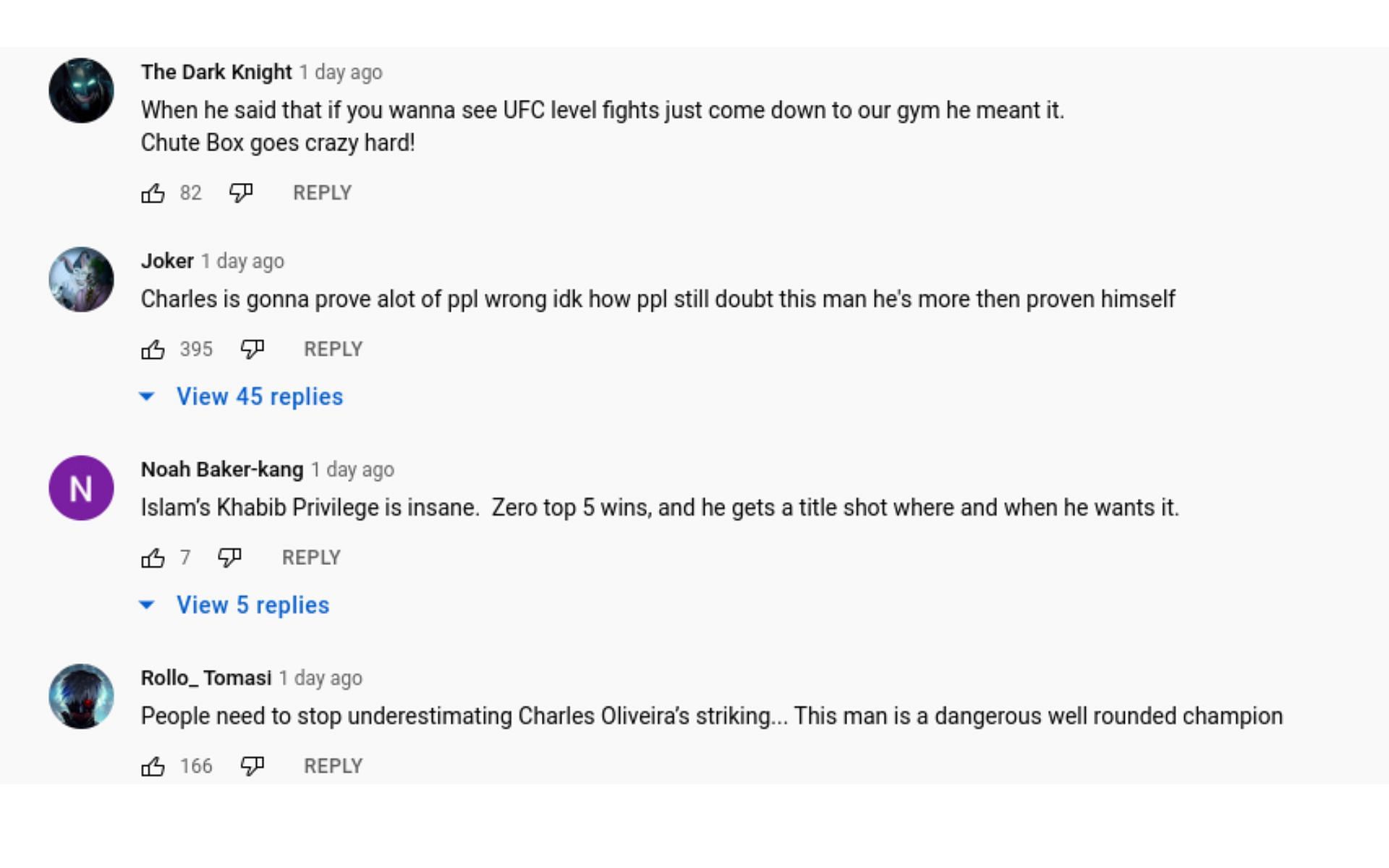The image features a striking portrayal of Batman, complete with glowing eyes, from a post made one day ago. The caption above the image reads: "When he said that if you want to see a UFC-level fight, just come down to our gym, he meant it. Shoot box goes crazy hard." This post has garnered 82 likes and no dislikes, with an option to reply located to the right of the like and dislike buttons.

Below this, there's a comment from a user named Joker, also posted one day ago: "Charles is gonna prove a lot of people wrong. I don't know how people still doubt this man. He's more than proven himself." This comment has received 395 likes and has prompted 45 replies, indicating a significant amount of engagement from the community.

Another comment from Noah Baker, marked by a purple circle, reads: "Islam's Khabib privileges are insane. Zero top five wins, and he gets a title shot when he wants." This one has a relatively lower engagement, with 7 likes and 5 replies.

Lastly, a comment from Thomas Rulo states: "People need to stop underestimating Charles Oliveira's striking. This man is a dangerous all-around champion." This comment has accumulated 166 likes and has 5 replies.

The background of the interface is a light gray, with various user pictures and interactive elements such as "like," "reply," and collapsible reply threads in blue, enhancing user engagement and discussion about UFC-related topics.